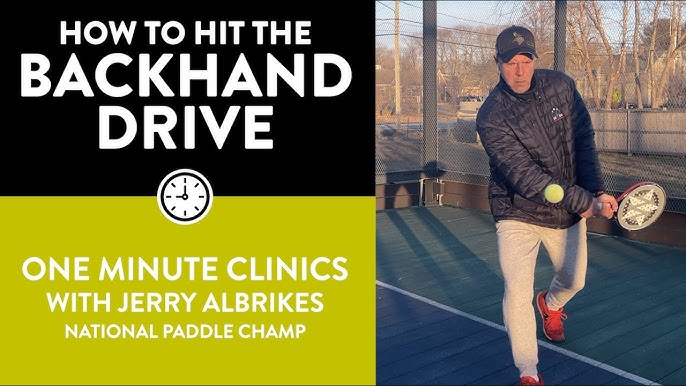This image is a detailed advertisement split into two sections. The left side has a black upper half transitioning into a chartreuse lower half. At the top, in bold white letters, it reads "How to Hit the Backhand Drive". Below this, in smaller white text against the chartreuse background, it states "One Minute Clinics with Jerry Albrecht's, National Paddle Champ". Between these sections, there's an analog clock set at 9 o'clock.

On the right side, the man identified as Jerry Albrecht, the National Paddle Champ, is captured mid-action on a paddle ball court. He is wearing a black puffer jacket, gray sweatpants, a black baseball cap, and red sneakers. He exhibits a focused expression as he hits a yellow ball with a paddle that has a star design. Behind him, the environment suggests winter, with bare trees and a wooden fence enclosing the court. The court itself has a green surface with white lines, indicative of a typical tennis or paddle ball court.